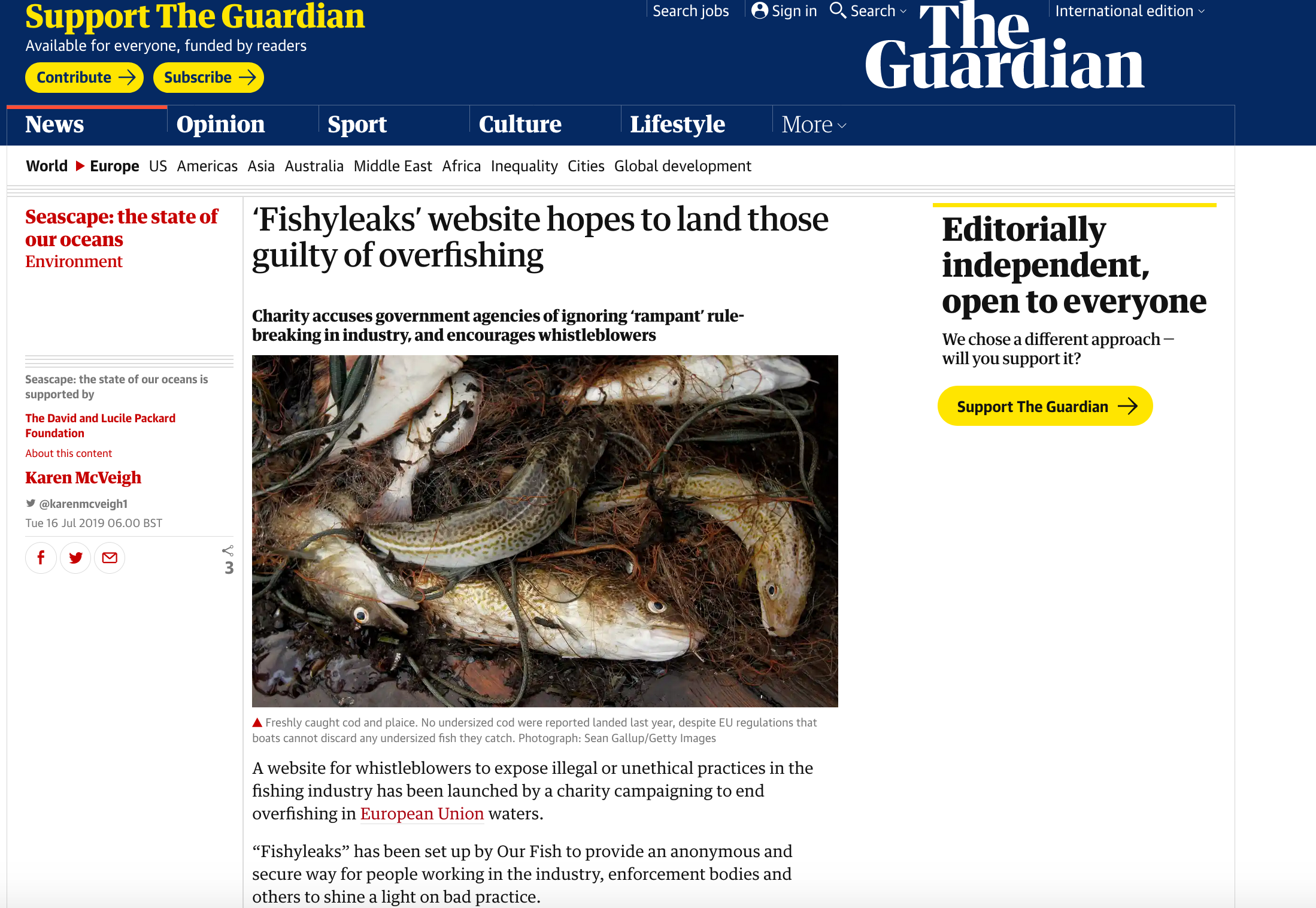The image depicts a page from The Guardian's website. In the top left corner, highlighted in yellow, there is a message saying "Support The Guardian" accompanied by a yellow "Contribute" button and a "Subscribe" button. The banner emphasizes that the content is "Available for everyone, funded by readers." Various sections such as News, Opinion, Sport, Culture, Lifestyle, and more are listed as clickable headings for easy navigation.

The featured section on the left, marked in red, reads "Seascape: The State of Our Oceans, Environment." To its right, the headline "Fishy Leaks: Website Hopes to Land Those Guilty of Overfishing" is prominently displayed. Below this headline, an image shows a disturbing scene of multiple fish ensnared in a fishing net, highlighting the grim reality of overfishing.

Below the image, an article is slightly visible, with the text indicating that the "Seascape: The State of Our Oceans" initiative is supported by the David and Lucile Packard Foundation. The article, written by Karen McVie, focuses on a new website designed for whistleblowers to expose illegal or unethical practices within the fishing industry.